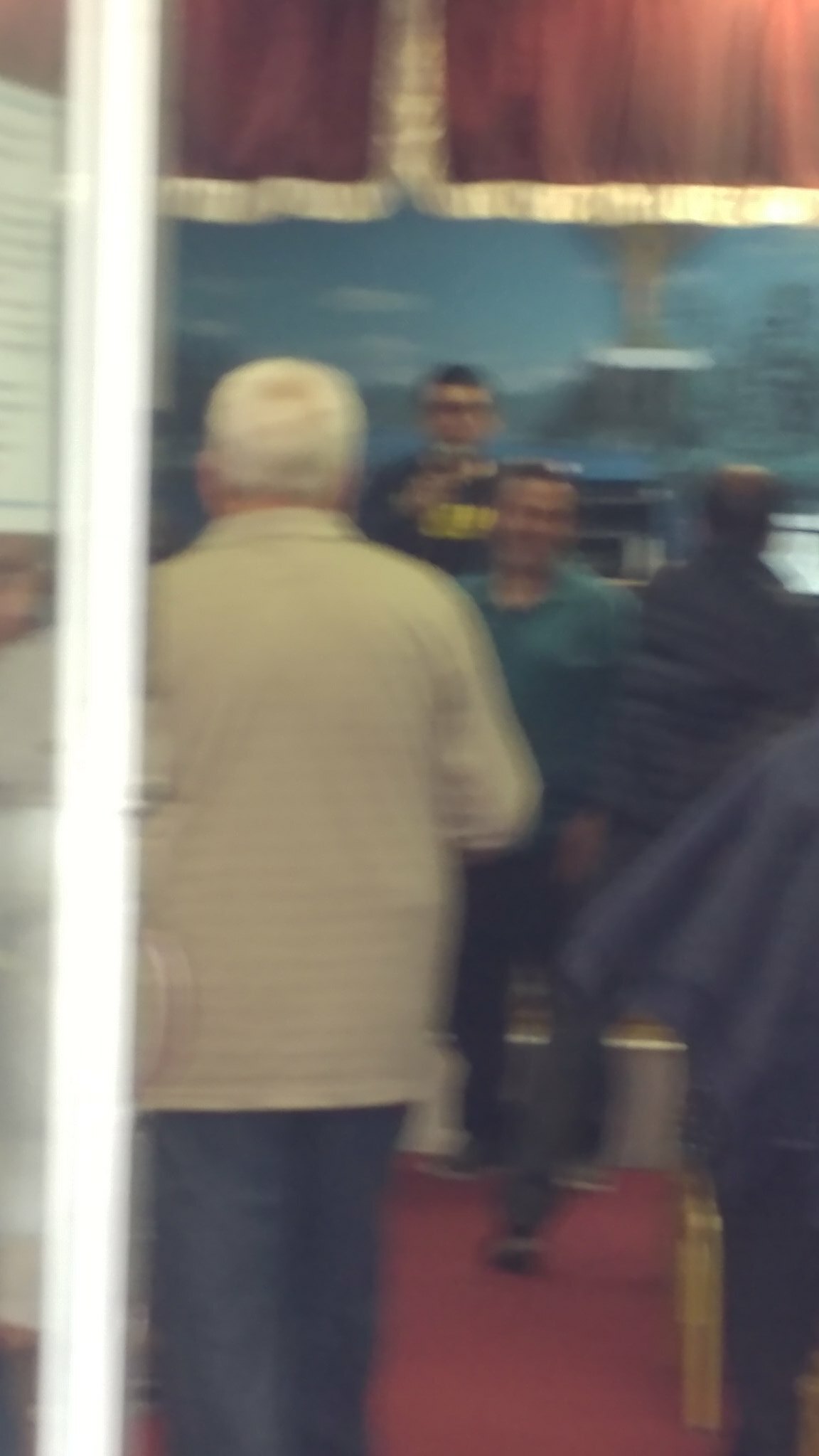This is an outdoor color photograph, presented in a vertical rectangular format that is significantly taller than it is wide. The entire image is out of focus, creating a blurry and indistinct scene. Dominating the left side of the frame, an older man with white hair is seen from behind, wearing a light-colored shirt or jacket and dark pants. Adjacent to him on the extreme left edge of the photograph is a barely visible white outline of what appears to be a glass door. 

To the man's right, there are three indistinct figures, one of whom seems to be moving towards him. This individual, possibly smiling, is dressed in a dark green shirt and dark pants. The setting features a red floor and is adorned with red curtains that have a gold border running along the top, contributing to an impression of an indoor establishment, perhaps a theater or a formal venue. Despite the lack of focus, the photograph evokes a scene of interaction within a structured space.